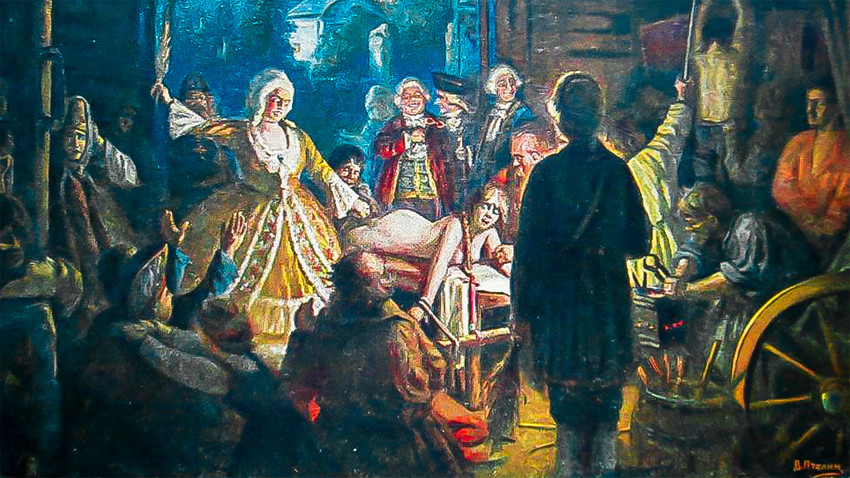In a vividly colorful, landscape-oriented painting reminiscent of colonial times, a dramatic and unsettling scene unfolds featuring numerous aristocrats adorned in opulent fineries. At the center, a naked young woman lies on her chest, strapped to a wooden table with her hands bound, her long ponytail cascading to the right. Her position and expression imply distress, as if impending harm were near. Dominating the left side of the scene, a woman dressed in a voluminous yellow gown and white wig holds a feather or branch in her raised right hand, poised over the prone figure as if ready to strike.

A backdrop of several men, garbed in attire akin to the Revolutionary War era, frames the scene. One man, distinguished by his red robe draped over a blue and yellow shirt and gray pants, smiles sinisterly from the background. To his right stands another man in a black hat, and further right, a third man clad in a blue coat and white wig. Additional observers, some appearing amused or entertained, populate the scene.

In the foreground, a large brown wagon wheel lies at the bottom right, juxtaposed with a barrel filled with ominous implements, perhaps knives or other tools. A man above this wheel grasps a pair of pliers, adding to the scene's tension. The setting appears barn-like, with a faint blue hue suggesting nighttime and an outdoor visage of trees and a building visible in the distance, enhancing the painting’s eerie atmosphere.

Overall, the painting captures a grim tableau where aristocratic figures witness the plight of a restrained woman, poised either to be whipped or subjected to a more severe punishment.